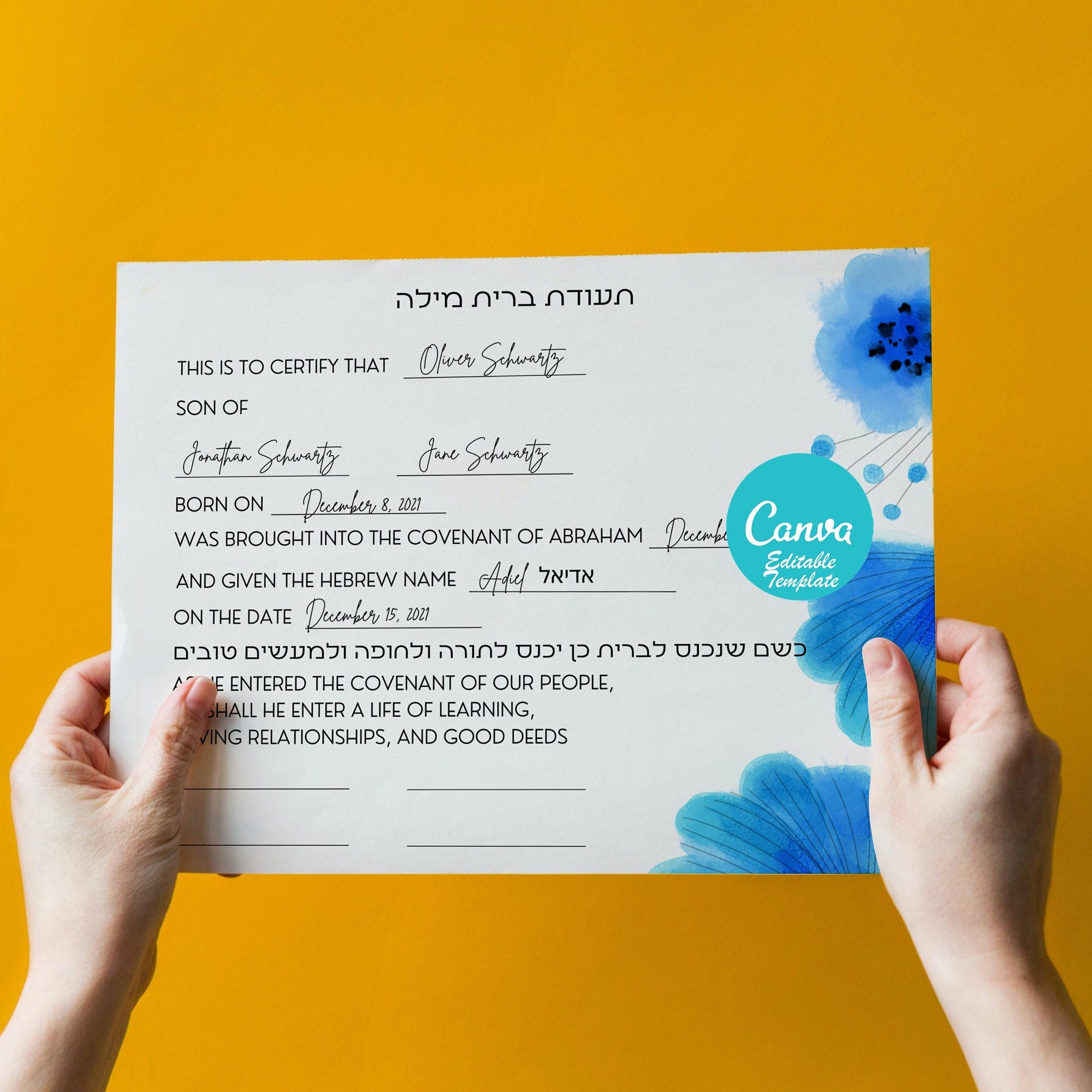The image features a certificate with a yellow background held by two hands, with only the hands, wrists, and a small portion of the arms visible. The certificate is partially covered by a light blue, teal-like circle with white text that reads "Canva Editable Template." The certificate contains both English and Hebrew text. At the top, it says in all caps, "THIS IS TO CERTIFY THAT," followed by the name "Oliver Schwartz, son of Jonathan Schwartz and June Schwartz." He was born on December 8, 2021, and brought into the covenant of Abraham in December 2021. The specific date can't be read due to the circle overlay. The text also notes that he was given the Hebrew name "Adiel" on December 15, 2021, with the date repeated in another line of Hebrew text. At the bottom, covered partially by the person's finger, it mentions that he "entered the covenant of our people, a life of learning, relationships, and good deeds." On the right side of the certificate, there are three blue flowers, with the top flower adorned with black specks.